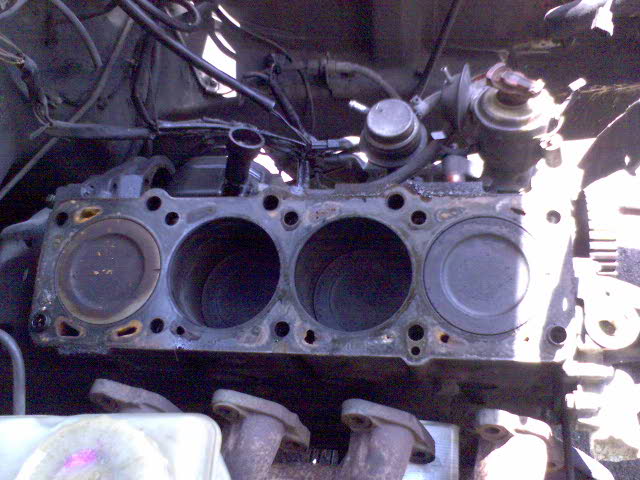The photograph captures a detailed close-up of a weathered, gray, and dirty industrial engine, likely belonging to a car or truck, situated outdoors. Central to the image is a large metal frame, possibly corresponding to the engine block, where the pistons would normally operate. Two of the piston chambers in the center are empty, suggesting the pistons have been removed or are missing, while the two outer chambers still contain metal round pistons. Above this assembly, several wires and cables connect to a circular metal piece, though it isn't attached to anything else, indicative of ongoing engine work or disassembly. Both air intake and gas intake pipes are visible, along with an electrical harness, hinting at potential repairs or modifications. The engine components exhibit a dark reddish steel color with scattered rust spots, emphasizing its old and well-used condition. The open hood allows sunlight to flood the scene from the right, creating high-contrast areas with some sections nearly blown out, whereas other parts remain in shade but still discernible. The bottom of the frame showcases thick metal coming to a rounded or pointed edge, extending outward and downward to form a diamond shape, completing the intricate and heavy-duty appearance of the engine.